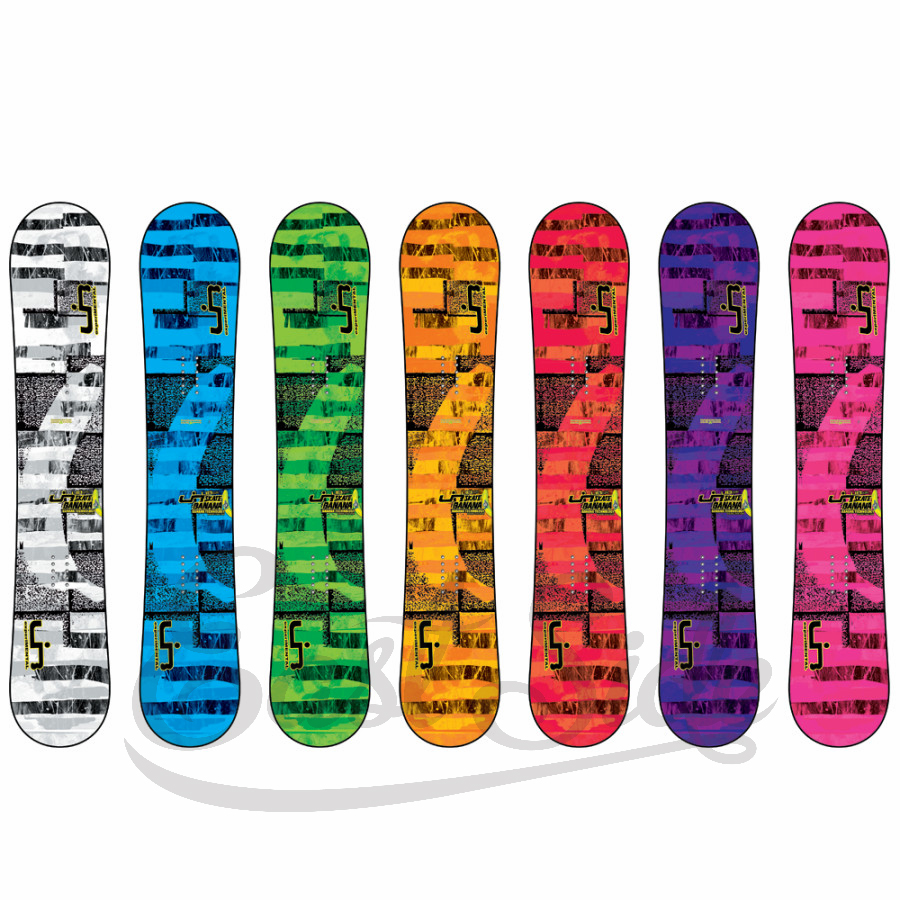The image illustrates a detailed, computer-generated lineup of seven skateboards, each showcased from a top-down perspective without wheels, set against a white background. These skateboards are uniformly designed—featuring dark gray line patterns, a faint number 7 embedded within the graphics, and a 'number 5' printed on both the top right and lower left corners. The graphics also include a swirled, faintly readable logo and the brand name "Skate Banana" alongside a small yellow banana icon centered on each board. The colors vary sequentially from left to right as follows: the first deck is predominantly white and gray, the second is medium blue and gray, the third is bright green and gray, the fourth is orange and gray, the fifth is pink and gray, the sixth is purple and gray, and the seventh is fuchsia and gray. Spread horizontally, these variations are likely displayed to assist potential buyers in selecting their preferred color. The detailed illustration, possibly an advertisement, is complete with a subtle watermark, indicating its origin from an online retail website.